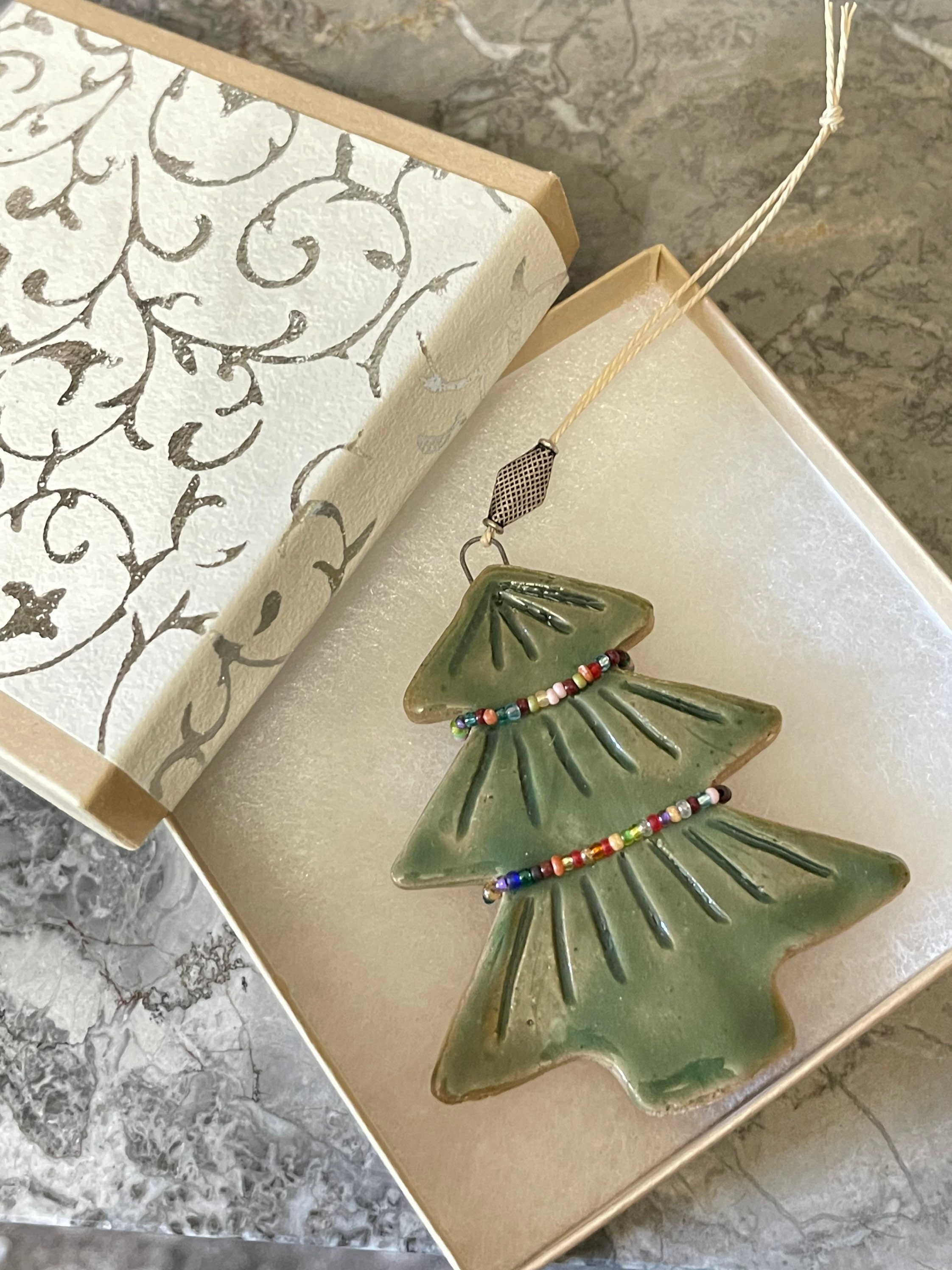This detailed product image showcases an ornamental pendant resembling a crafted Christmas tree, elegantly placed inside a shallow, open tan gift box with silver filigree embellishments on its exterior. Resting on a padding of foam within the box, the pendant embodies a three-tier clay Christmas tree, reminiscent of a cartoon depiction, featuring three stacked triangle layers. Painted and glazed in a vibrant green, the tree is adorned with tiny, colorful beads—blue, turquoise, red, gold, and green—strategically placed around its cinched widths to emulate festive ornaments or lights. At the tree’s top, a clasp secures an off-white handmade string hanger, facilitating easy display. The setting is atop a sleek marble or quartz surface, viewed from above, presenting a clean, indoor scene without any intrusive text or additional objects, thereby emphasizing the tree's intricate details and festive charm.